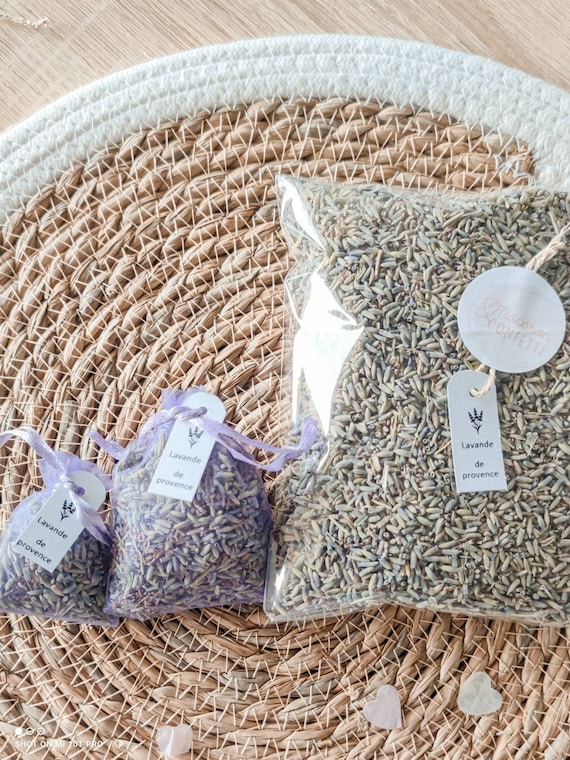The image depicts a detailed product display of three plastic bags placed on a woven circular placemat with a beige wood backdrop. Each bag is tagged with cardboard labels tied with twine, inscribed with "Lavande de Provence" in black text, indicating they contain lavender products. The placemat features intricate weaving resembling bamboo with a geometric triangular pattern, enhancing the rustic aesthetic. The left and middle bags are medium-sized, encased in a translucent lavender-colored layer, and adorned with purple ribbons. The larger bag on the right contains green, seed-like items, and is also labeled. White hearts and small lavender sprigs add delicate embellishments to the scene, while white stickers or labels are visible on the packaging. The arrangement forms an appealing and carefully curated display, highlighting the handcrafted and aromatic qualities of the lavender products.